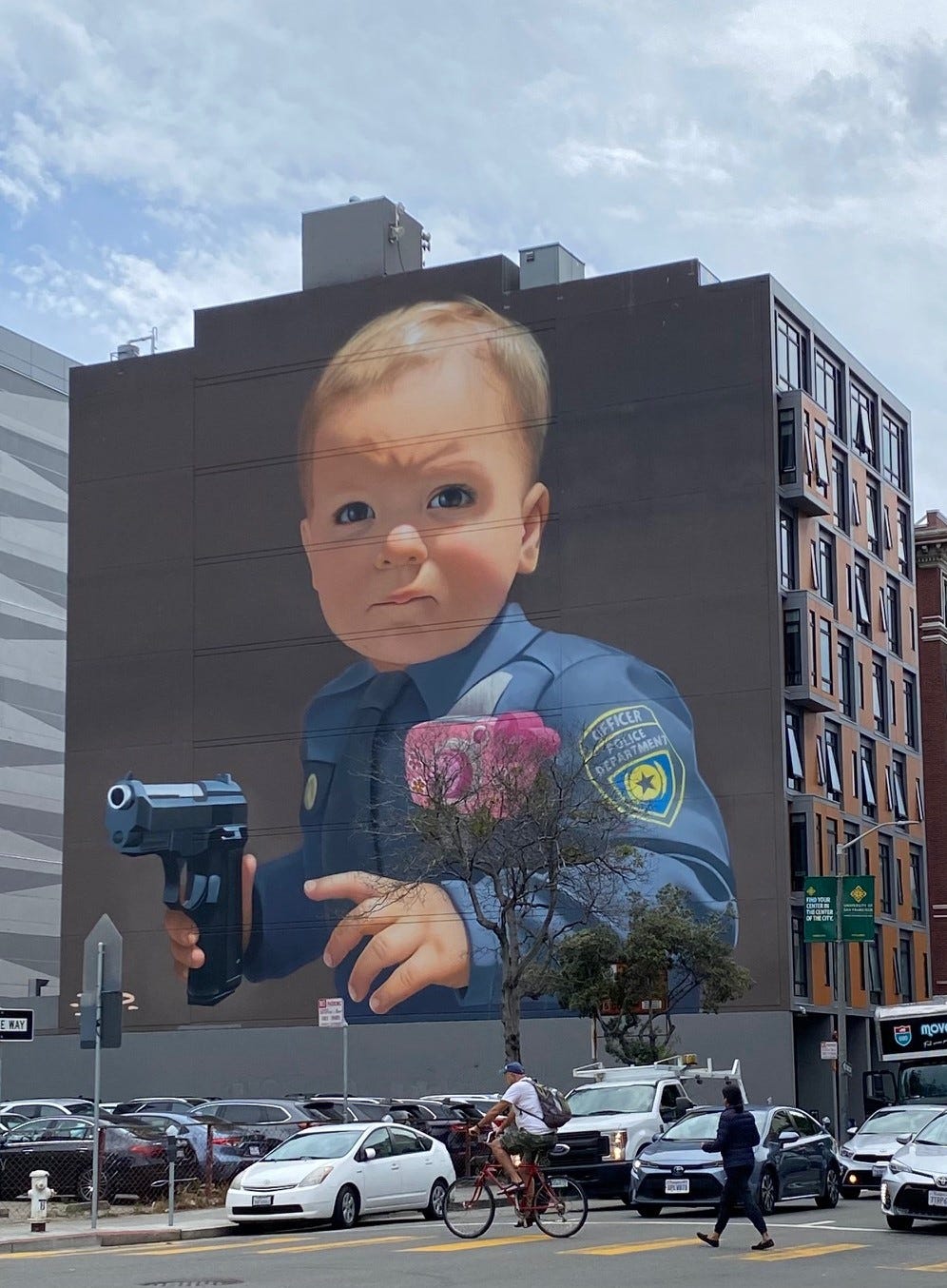This image depicts a vibrant urban scene captured during a clear daytime, with a blue sky dotted by fluffy clouds. The focus is a seven-story city building with a striking mural covering the entire side. The mural showcases a toddler-aged child with short blonde hair dressed in a blue police uniform, complete with a dark blue tie and a patch on the left arm labeled "Officer Police Department" with a yellow circle and blue star insignia. The child is holding a handgun in their right hand and has a pink, childlike camera mounted on their chest. The mural side of the building, unlike the rest which features numerous windows—some slightly open and in lighter shades of brown—has no windows. Below, a busy street scene includes pedestrians walking, a cyclist, and several cars both parked and in transit. The building stands beside a parking lot filled with vehicles, reinforcing the bustling city atmosphere.